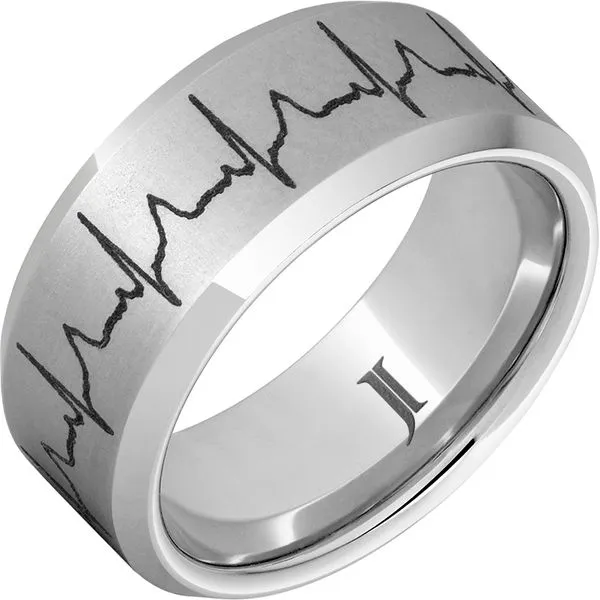The image depicts a sleek men's engagement ring made of titanium, characterized by its shiny, silverish metal surface that is clearer and less cloudy than silver. The ring features rounded beveled edges that taper inward. On the exterior, a repeating heartbeat pattern—similar to a heart monitor or lie detector line—has been laser-etched in black, adding a touch of modern elegance. Inside the ring, the initials "JL" are engraved back-to-back, also in black, signifying a personal touch. The overall design combines durability with intricate details, making it a unique symbol of commitment.